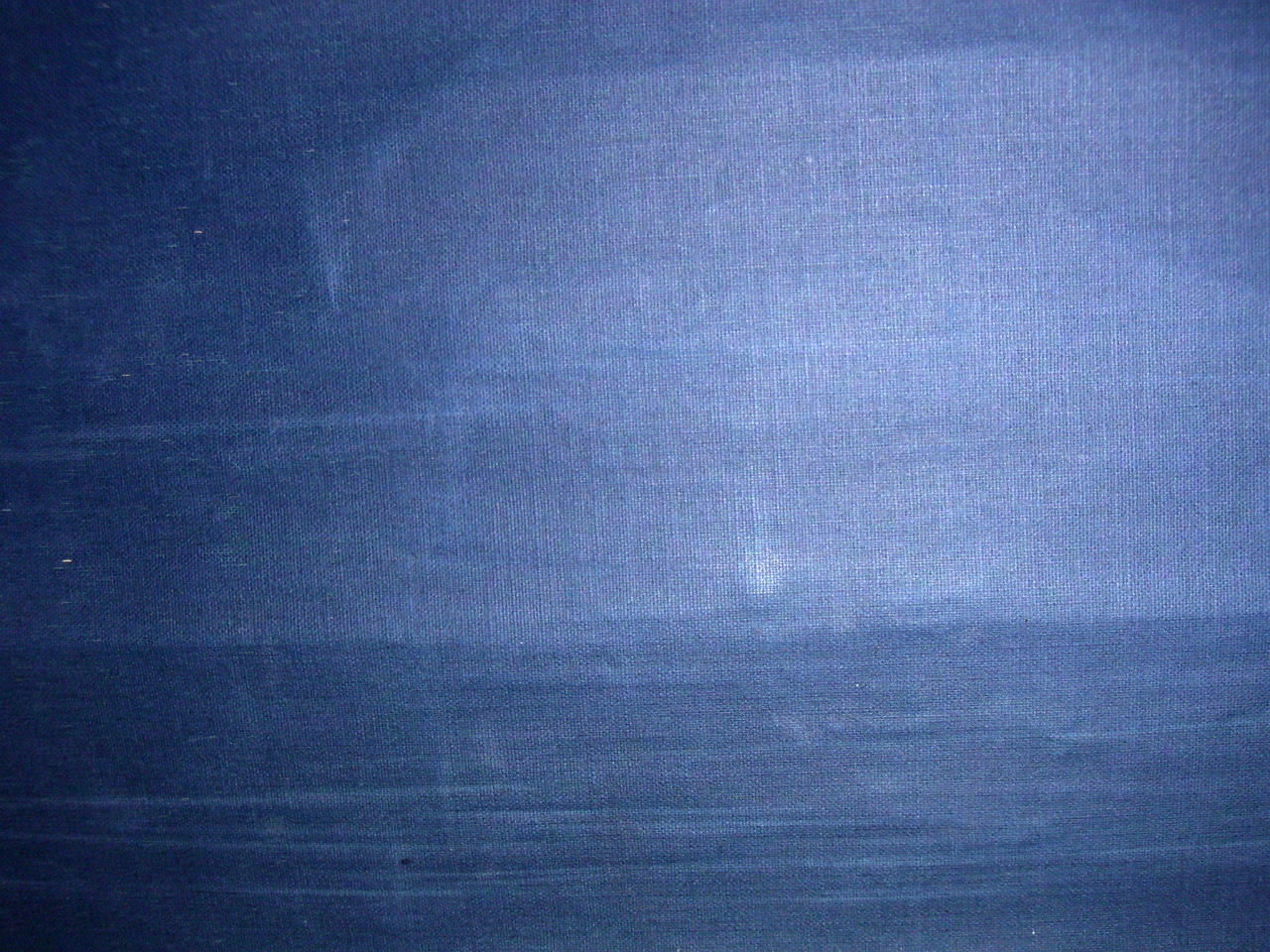The image features a close-up view of a dark navy blue vinyl fabric, commonly seen on items like outdoor umbrellas, tablecloths, or vehicle covers. The fabric exhibits a glossy finish with noticeable scuff marks, making certain areas appear lighter. The image is tightly focused, showing the material wrapped snugly around an unidentified object, with some tension points creating distinct shapes: a hanging V shape towards the top left and a small circular protrusion near the center. The blue hue is consistent across the surface, interspersed with thin white streaks and specks—likely imperfections or dust particles. The lighting appears more intense at the center of the image, gradually dimming towards the edges, giving a subtle gradient effect. These details suggest a high level of magnification, capturing both the texture and minor flaws of the vinyl fabric.